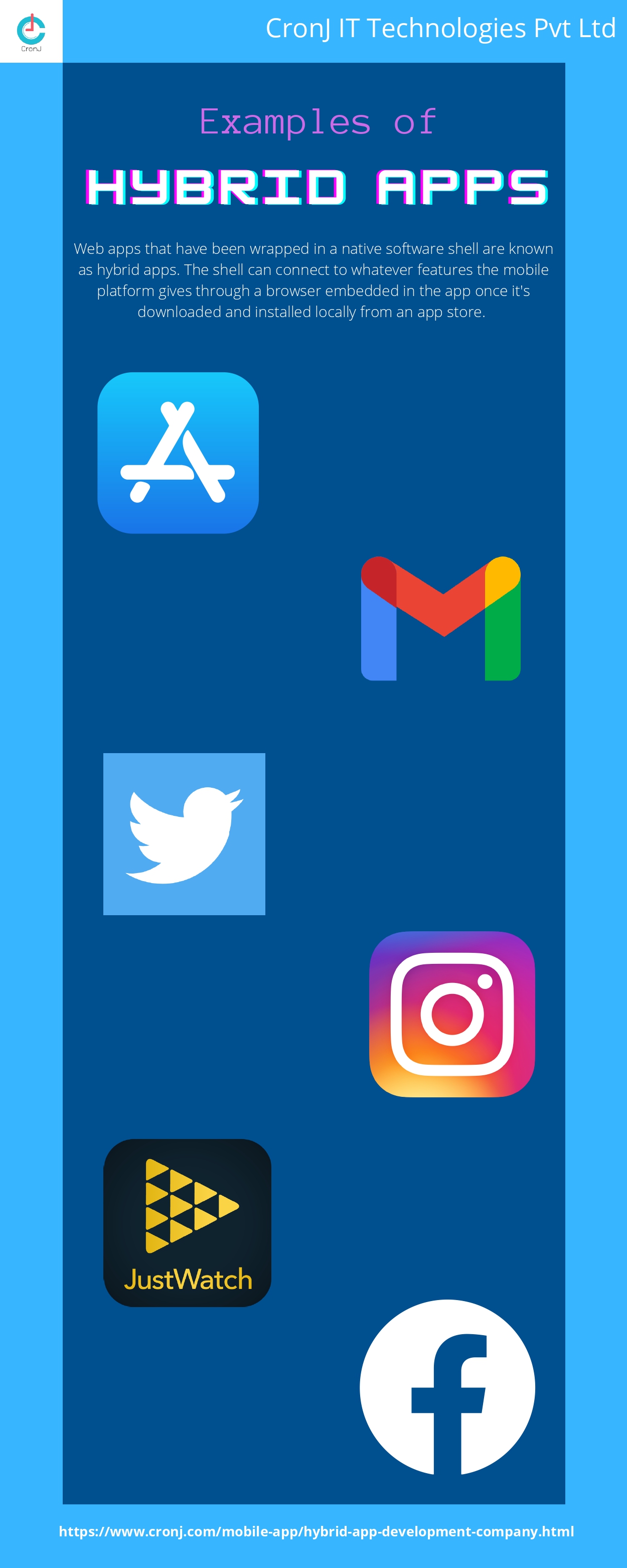The image displays an informational sheet with a prominent dark blue rectangle centered against a light blue border. In the top left corner, within a small white square, there is a logo featuring a letter 'C' with two clock hands—one pointing up and the other to the left. Below the 'C' logo, there is some indistinct text. The top right corner of the sheet features the text "Cronge IT Technologies Private Limited." At the bottom of the sheet, a link to the company's website is provided. 

Within the central dark blue rectangle, the heading reads "Examples of Hybrid Apps." The main text explains that "Web apps have been wrapped in a native software shell that are known as hybrid apps. The shell can connect to whatever features the mobile platform provides through a browser embedded in the app once it is downloaded and installed locally from an app store." 

Below this explanatory text, there are icons representing various apps, including Gmail, Twitter, Instagram, and Facebook, illustrating examples of hybrid applications.